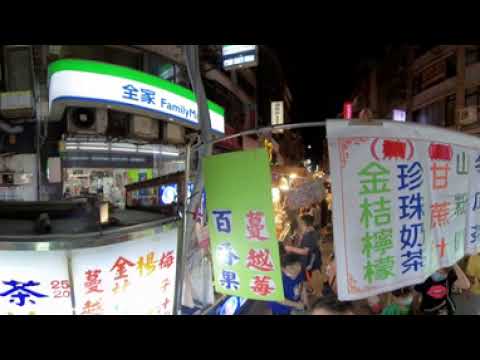This low-resolution, photorealistic nighttime image captures a bustling outdoor market or shopping center, likely in an Asian country, given the numerous banners with Asian characters. The scene is viewed from an aerial perspective, showcasing a crowded walkway flanked by stalls or shops. The walkway is partially obscured by various signs; a bright green one with blue and red characters hangs centrally, while a white sign featuring green, blue, red, and orange characters is on the right.

The area is well-lit despite the dark, black sky, indicating it is night. Tall brown buildings surround the walkway, with one on the left prominently displaying a large, illuminated white and green sign with English and Asian writing. This sign includes the partial English word "family" and the numbers 25 and 20. Visible air conditioning ducts on some shops give an impression of a bustling environment where vendors and shoppers are engaged in vibrant activity. Although individual items or shops are hard to make out, the overall scene conveys a lively nighttime market atmosphere.